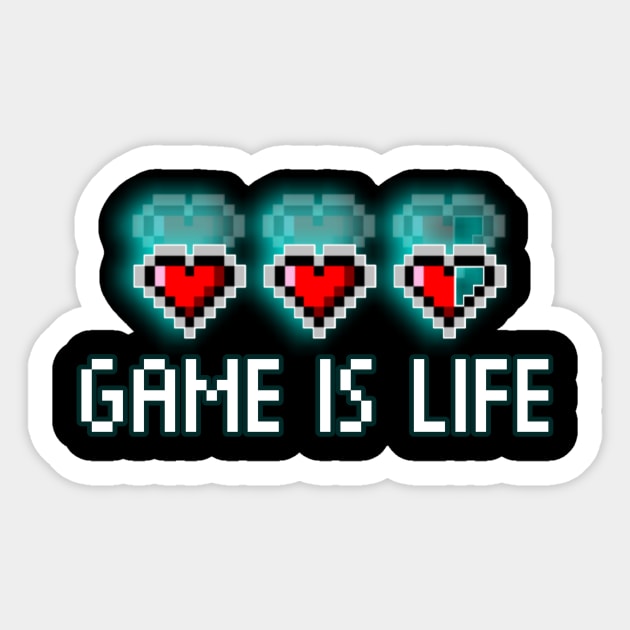The image depicts a sticker or poster set against a light gray background, bordered by a thick white perimeter. Central to the design is the phrase "GAME IS LIFE" rendered in pixelated white font over a black background. Above the text, three pixel art hearts are displayed, resembling those commonly used to indicate a player's health in retro video games. Each heart is designed using pixel blocks, with the first two hearts fully red, symbolizing full life, while the third heart is half red and half green, signifying two and a half remaining lives. The detailed pixelation and nostalgic design evoke imagery from classic 80s video games.